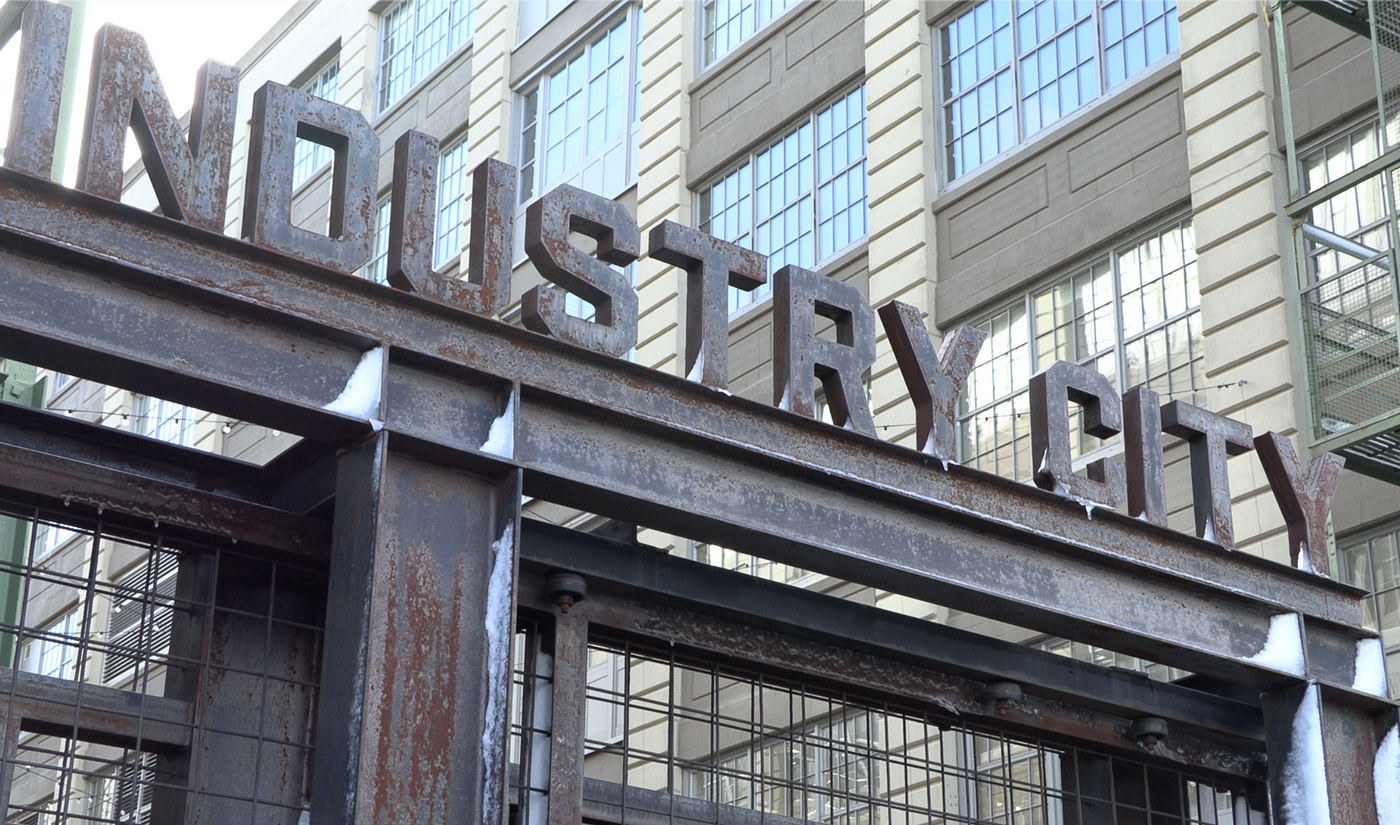A detailed zoomed-in image of an exterior scene, focusing on a building and a sign. In the middle-right area of the image, there's a building composed of distinct sections. One section is white and rectangular, displaying a patterned design. Adjacent to it are windows segmented into three parts, each part containing multiple small rectangles outlined in gray. Below the windows, the pattern continues with more gray elements. A rusted sign with silver and reddish-brown corrosion reads "INDUSTRY CITY" in bold capital letters. The lower portion of the image includes a partial view of a fence with visible squares and bars, though the full structure and what's beneath it are obscured.